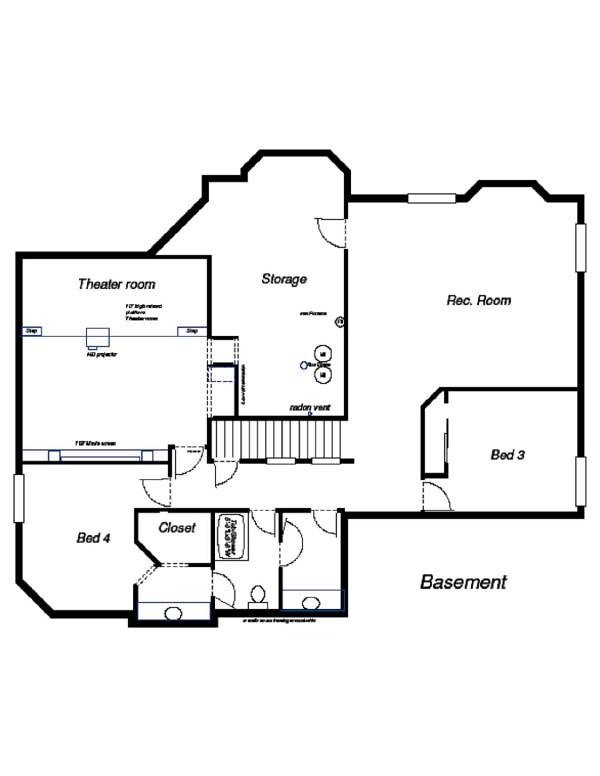This blueprint features a detailed layout of a residential floor plan. To the left, there is a fully-equipped theater room, complete with an HD projector. Adjacent to this, on the right, is a storage area, which then leads into a spacious recreation room. Directly connected to the recreation room is Bedroom 3, situated further to the right. Moving left from Bedroom 3, there is an open room, the purpose of which is not specified. Next to this open area is another room, likely a bathroom, with a closet adjoining its left wall. To the far left of the plan, you will find Bedroom 4, which also seems to have an attached bathroom. The layout clearly indicates the direction of door swings throughout the floor plan. Additionally, the basement is located on the far side, just outside Bedroom 3.